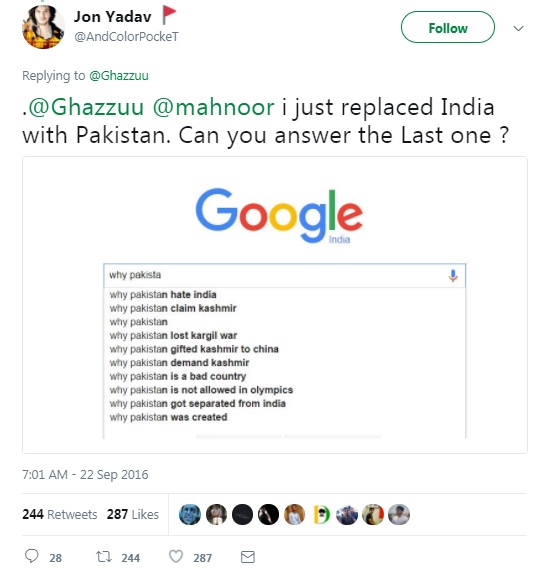Here's the cleaned-up and detailed caption:

---

In this image, we see a screenshot, apparently taken at 7:01 a.m. on September 22, 2016. The image features a tweet from a user with the display name "John Yadav" (spelled as John Yad av or Yadav), who has a red flag icon next to their name. The tweet appears to be a reply to another user named @Ghazzuu, referencing a tweet from @GazooManor. John Yadav's tweet states, "I just replaced India with Pakistan. Can you answer the last one?" 

The screenshot captures a Google search result under "Google India," where someone has altered the query "Why India" to "Why Pakistan." The auto-complete suggestions now include a series of politically charged questions:

1. Why Pakistan hate India?
2. Why Pakistan claim Kashmir?
3. Why Pakistan in Ligur's war?
4. Why Pakistan gifted Kashmir to China?
5. Why Pakistan demand Kashmir?
6. Why Pakistan is a bad country?
7. Why Pakistan is not allowed in Olympics?
8. Why Pakistan got separated from India?
9. Why Pakistan was created?

These query suggestions reflect common questions around the India-Pakistan relationship and broader geopolitical issues, hinting at underlying tensions and curiosity surrounding these topics.

---